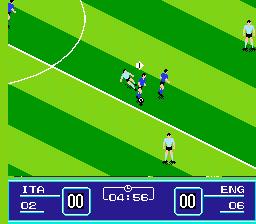This is a color screenshot from a mid to late 1980s video game, likely on a system like the NES or Sega Master System, featuring a soccer match between Italy and England. The graphics are primitive but advanced beyond simple stick figures, with players rendered in short black shorts, long white socks, and shirts—Italian players in blue jerseys and the English team in lighter-colored jerseys. 

The soccer field is depicted with alternating dark and light green stripes, simulating a freshly mowed field, and the scene centers around midfield within the center circle. Several players are visible: three in light blue near the center, five in darker blue surrounding the soccer ball, and one of the lighter blue players kicking the ball. 

At the bottom of the screen, a blue bar indicates the score: ITA 0-2 and ENG 0-6, with the actual score appearing as 0-0. A clock icon shows 4 minutes and 56 seconds have elapsed in the game. An additional detail includes an arrow pointing to the right beside a player in a white jersey, emphasizing their current direction or action in the game.